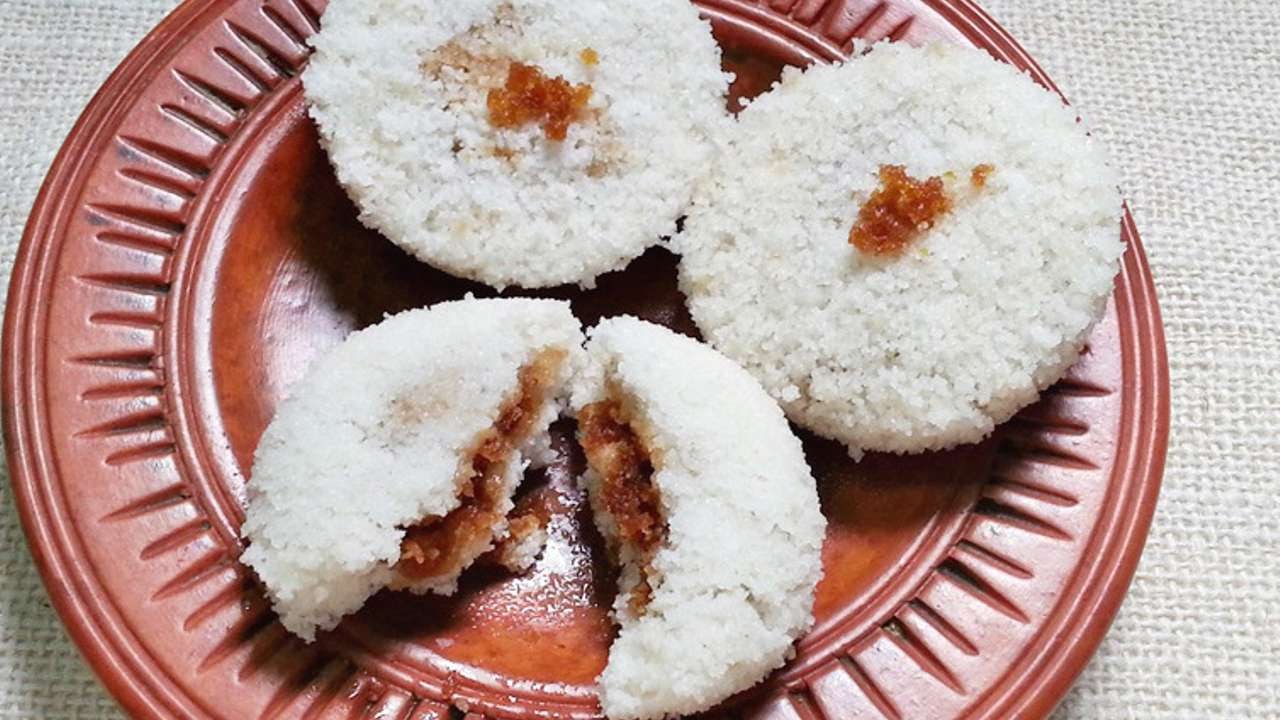The photograph, taken indoors, showcases a detailed top-down view of three circular, white pastries displayed on a decorative reddish-rust plate. The plate features a depressed center and indented circular outlines with vertical stripes around the edge. One pastry is broken open, revealing a reddish strawberry-colored filling, while the other two remain intact, their crumbly exteriors dusted possibly with powdered sugar. The pastries might be cookies, filled mochi, or donuts, with textures suggesting a rice covering or delicate crust. They sit on a thick, cream-colored woven tablecloth, adding a cozy touch to the presentation. The composition highlights the intricate design of the plate and the subtle contrasts in texture and color between the pastries and their setting.